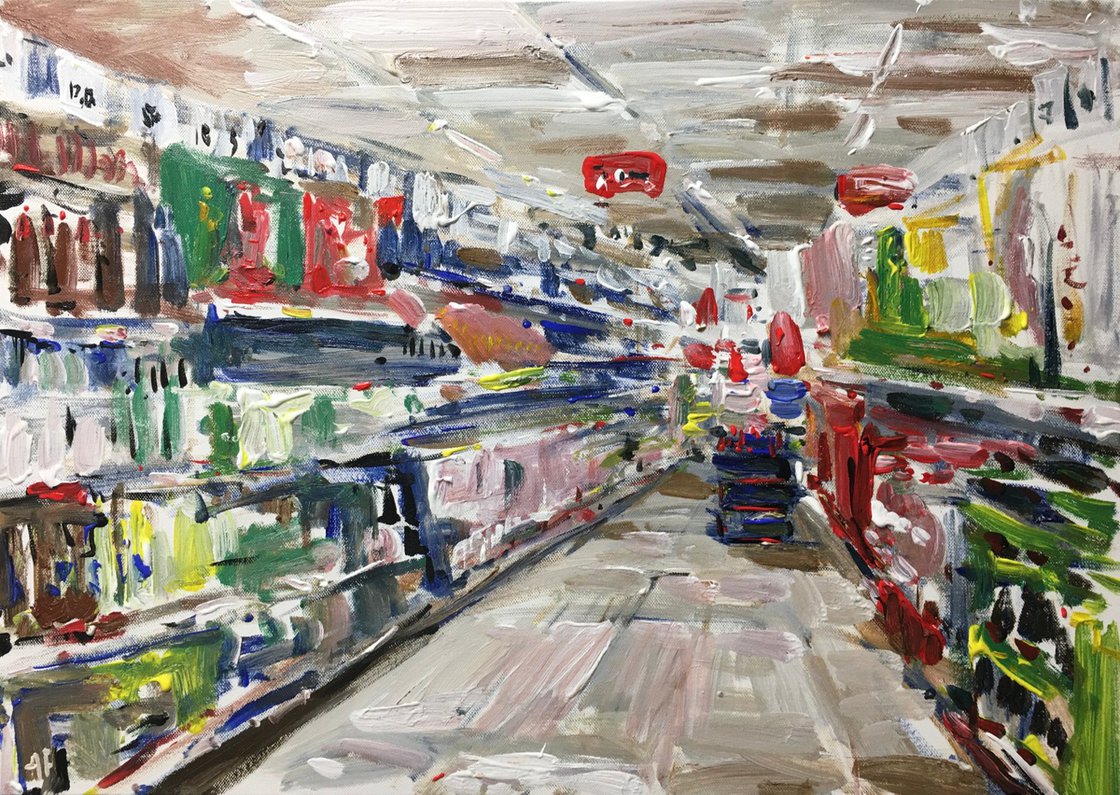This image is an abstract, Expressionist-style painting titled "Supermarket," created using a combination of palette knife and thick brushstrokes, making the rich texture and thickness of colors apparent. The scene is set inside a store, with an aisleway leading between two sets of shelves that extend from the bottom edges of the painting towards the center. A pathway, depicted with grey tile flooring, runs down the middle. At the end of this aisle, there is a blue cart and what appears to be a display featuring stacked shirts hanging from a mannequin.

The items on the shelves are varied and colorful, with objects on the left in reds, greens, pinks, and yellows, possibly representing kitchenware or cans. On the right, the objects include bags, boxes, and maybe even clothing. Despite the diversity of items, the details are blurred and run together, characteristic of the Expressionist style. The store scene is framed by a ceiling rendered in a glossy, creamy white with red fire detectors. A prominent red box hangs from the ceiling, adding to the modernist color scheme of reds, greens, browns, blues, and whites. The overall image, though detailed and elaborate, remains somewhat indistinct, emphasizing the abstract, impressionistic nature of the painting.